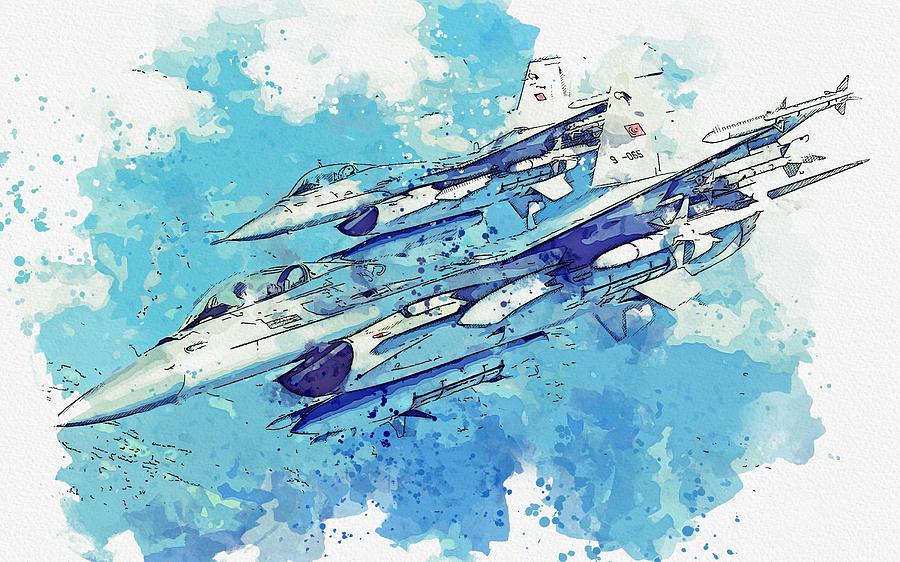This is an illustration that appears to show two fighter jets flying at high speed, heading downwards and to the left. The jets are adorned with large missiles on their wings and beneath them. The lower jet features a visible pilot and the number "9065" in black font near its tail. Above this, there is a flag emblem that is square, in a reddish or pinkish color with a crescent to the left, and an indistinct symbol in the center. The second jet also has a similar flag design, although less discernible, and no visible numbers. The backdrop of the image transitions from white at the edges to a splash of blue in the center, with darker blue at the bottom and an almost light blue teal at the top. The overall appearance suggests a hand-drawn style, likely mimicking a view from another aircraft. The entire scene is awash with overlapping hues of blue, light blue, dark blue, and white, which blend with subtle strokes of red and peach.